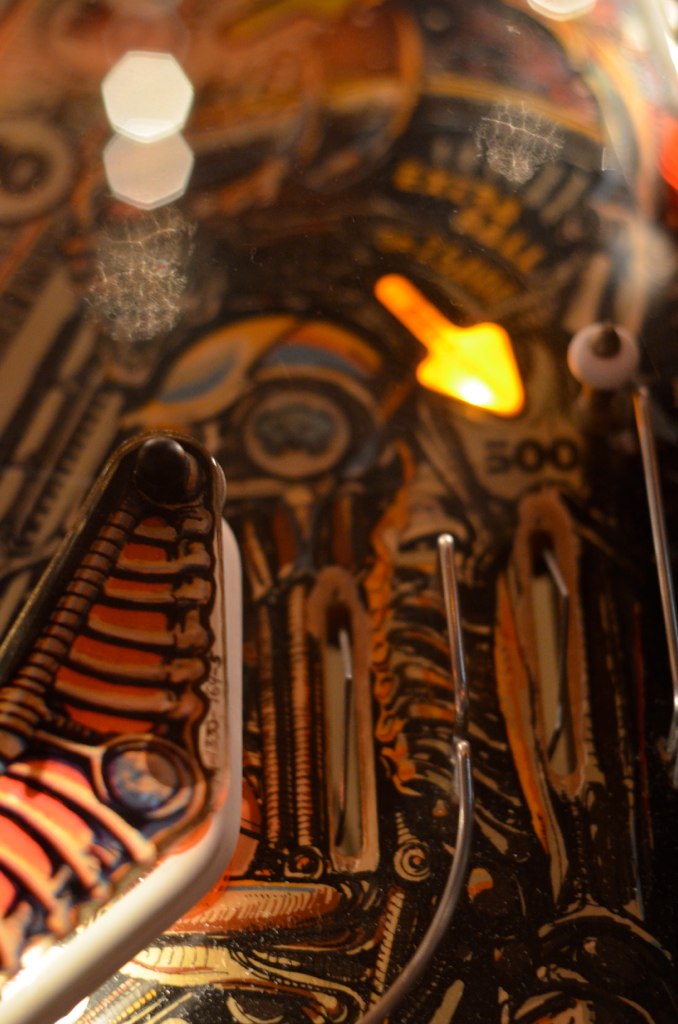This photograph, with a vertical rectangular alignment, captures a highly detailed and zoomed-in view of a pinball machine's intricate mechanics and artwork. The image is set indoors, possibly in an arcade or game room. At the center of the focus is a collection of silver levers and rails, interspersed with red elements and springs, creating what appears to be a path for the pinball. A prominent feature is a lit red arrow with a yellow tip, pointing downward to the right, and an unreadable text atop the arrow.

In the upper left-hand corner are two hexagonal shapes—one white and one light brown—blurred out slightly, contributing to the complex visual texture. Also noticeable is a white bumper, resembling a round washer typically found in pinball machines. Throughout the image, there are artistic elements that resemble bones, colored in orange with brown tips, and scattered across various components.

Though some parts of the photograph are slightly out of focus, the diverse color palette of black, white, yellow, orange, red, blue, and gray adds vibrancy to the scene. Despite the lack of readable text, the image vividly showcases the mechanical and artistic details that make up the pinball machine, creating a rich, dynamic, and immersive visual experience.